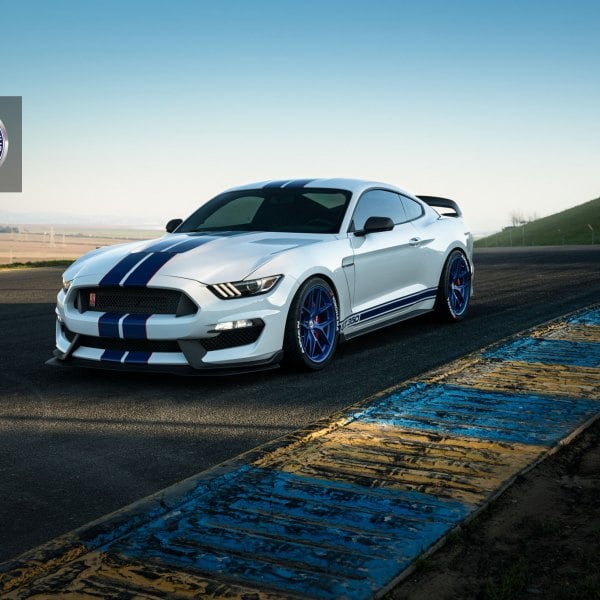This professional photograph captures a striking white Ford Mustang parked on a sunlit asphalt track, which features distinct blue and yellow borders signifying its edges. The sky above is a clear, cloudless blue, giving the scene a bright and open atmosphere. In the backdrop, there is a lush green hill covered in grass, while to the left, there appears to be either a beach or a field adding a touch of natural beauty to the setting.

The Mustang itself commands attention with its two bold blue racing stripes that run vertically from the front across the hood and roof. The car's aggressive stance is accentuated by a rear spoiler and its geometric, spoked blue rims. Adding a touch of character, the side of the vehicle features black banding with 'GT 350' graphics on the lower part of the passenger door. This two-door sporty vehicle, though not fully decked out, stands out with its blend of sleek design and racing elements. The black asphalt track beneath, coupled with the ribbed concrete strip in blue and yellow, gives it an authentic racing vibe, making it the focal point of this vibrant, daytime countryside scene.